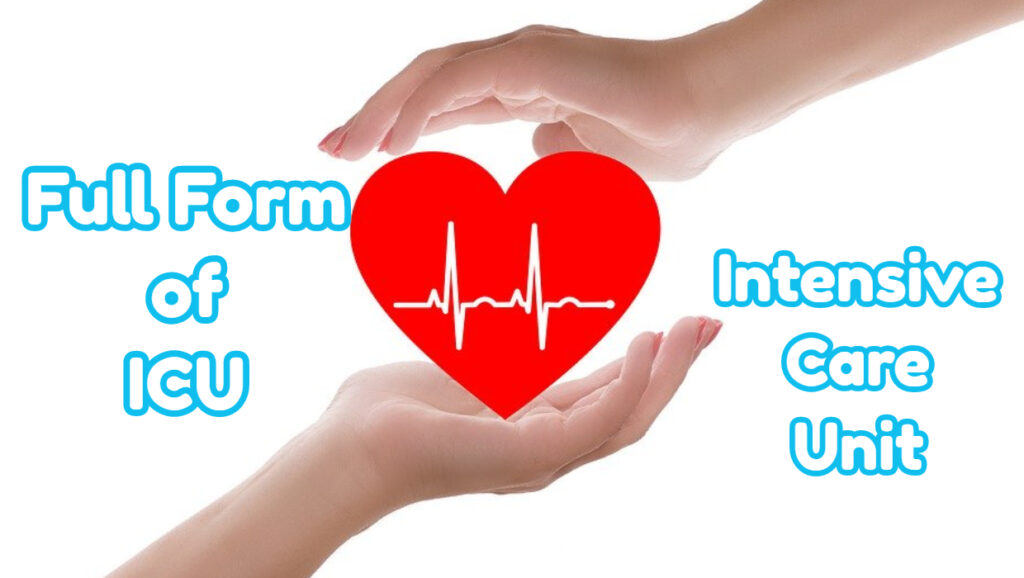The image features two Caucasian hands with a red heart between them on a white background. The hand from the bottom left is palm-up, while the hand from the upper right is palm-down, both positioned to cradle the heart in the center. The heart has a white EKG-like squiggly line inside, symbolizing a heartbeat on a monitor. On the left side of the heart, the phrase "full form of ICU" appears in three lines, centered, with white text outlined in blue. Similarly, on the right side, the words "intensive care unit" are arranged in three lines, also centered, with white text outlined in blue. The text style is rounded and slightly cartoony, contributing to the overall warm and caring theme of the image.